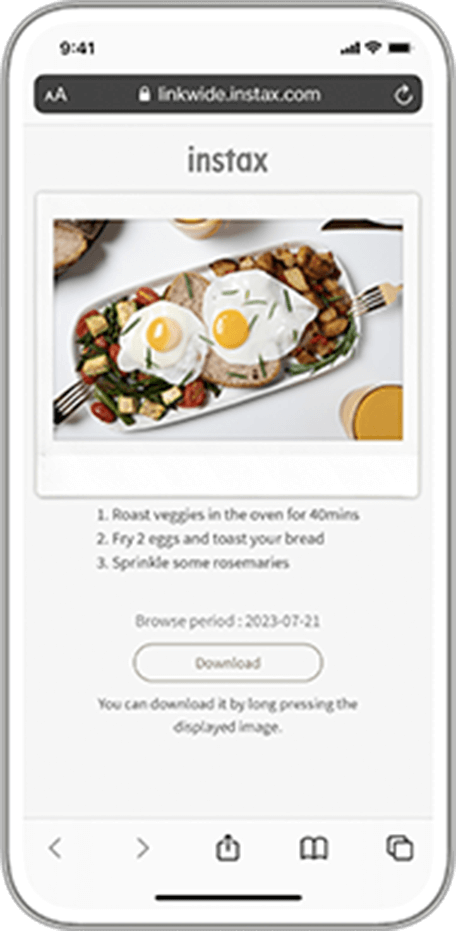The image displays a tablet screen showing the time as 9:41. The address bar at the top includes a lock icon followed by the URL "linkwide.instax.com," with a refresh button adjacent to it. Below the URL, the text "Instax" is prominently displayed. Further down, there is a box containing an appetizing meal setup: a large platter filled with a variety of foods. On the left side of the platter, there is a fresh salad adorned with tomatoes and croutons, accompanied by green beans and a slice of bread. The main section of the platter features two sunny-side-up eggs sprinkled with parsley, alongside some crispy fried potatoes. Silver forks are placed on both the left and right sides of the platter. To the right of the meal, an orange cup is visible. At the bottom of the image, there are cooking instructions listed: 
1. Roast veggies in the oven for 40 minutes.
2. Fry two eggs and toast your bread.
3. Sprinkle some rosemary.
A download button is also present, suggesting additional content or a recipe download option.